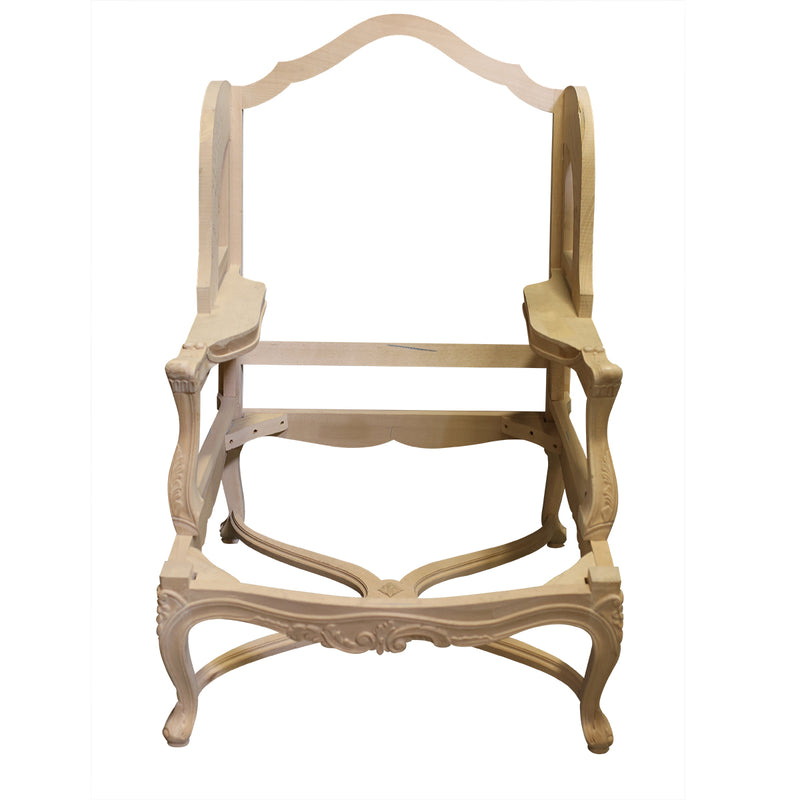The image depicts an ornate and intricately detailed wooden chair frame, emphasizing the craftsmanship and decorative elements. The light, white-washed hardwood is skillfully carved with intricate leaf designs that embellish the frame, particularly on the armrests, front panel, and legs, with the latter featuring animal foot designs at the base. The armrests are scalloped and adorned with additional carvings, seamlessly connecting to the back piece, which arches upward in an elegant curve resembling an 'N' shape. The frame reveals structural support in a square base, reinforced by an X-shaped brace, and is ready for reupholstery, missing its back, arm, and seat cushions. The overall condition appears excellent, indicative of sturdy construction and a design that likely draws inspiration from French furniture styles.